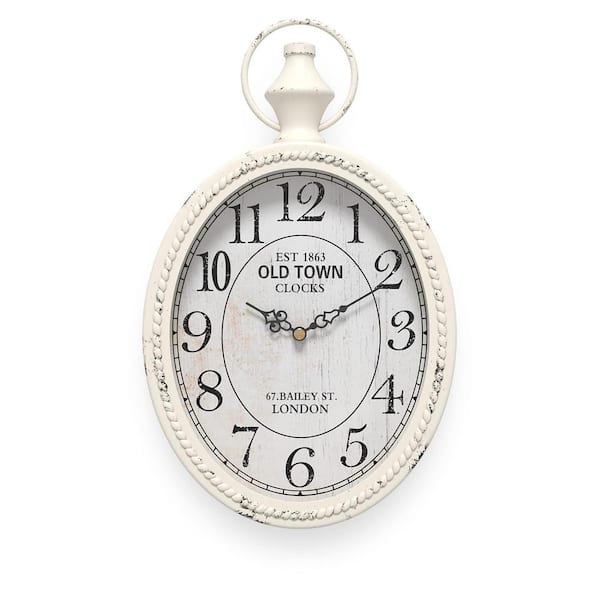This is a detailed color photograph of an antique-style clock designed to resemble a vintage pocket watch. The clock has an elongated oval face with a weathered white surface and black numbers. It features a braided rope-like frame, also white and distressed, suggesting an intentional aged effect. At the top of the clock is a winding knob with a metal hoop, indicating it could be latched onto a chain. The face of the clock has ornate hour and minute hands set to 10 and 2, held by a gold pin in the center. The numbers, from 1 to 12, are large and slightly curled. In the middle of the clock face, it reads, "EST established 1863, Old Town Clocks," with "67 Bailey Street, London" in smaller black lettering below. The background of the photograph is completely solid white, making the clock stand out prominently.